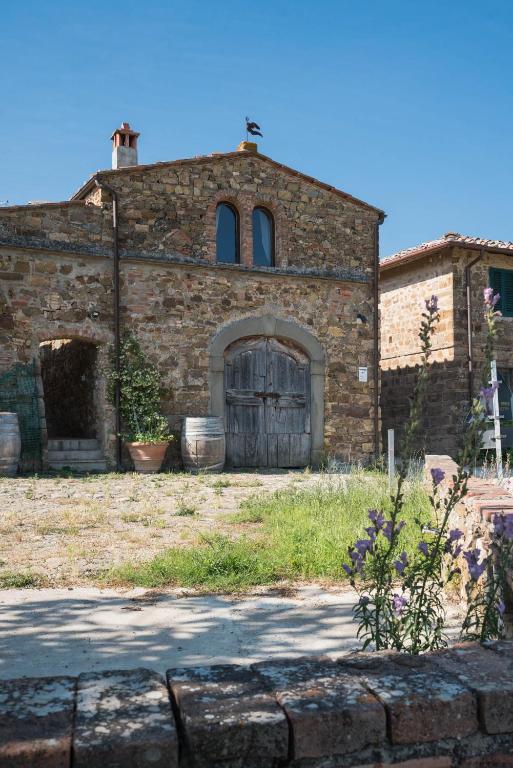The image captures an old, abandoned structure likely dating back to the late 1800s or early 1900s, reminiscent of Spanish architecture. The two-story building is predominantly constructed from stone with varying shades of brown, gray, and black. The facade features an imposing, arched wooden barn door composed of unmaintained wooden planks, flanked by two vertically rectangular windows with arched tops situated on the second level. On the left, a smaller, open doorway is accessible via three small gray steps.

The image is set against a backdrop of a clear blue sky, accentuating the building’s worn and rustic appearance. A patchy front lawn, with vibrant green grass on the right and sparse brown grass on the left, extends up to a small brick fence with purple blossoms peeking through. Beyond the brick fence, a narrow sidewalk runs parallel to the building. There is also a partial view of another structure to the right of the main building, suggesting a courtyard or possibly another section of the house, but the exact details remain obscured. The overall scene imparts a sense of historical charm amidst natural decay.